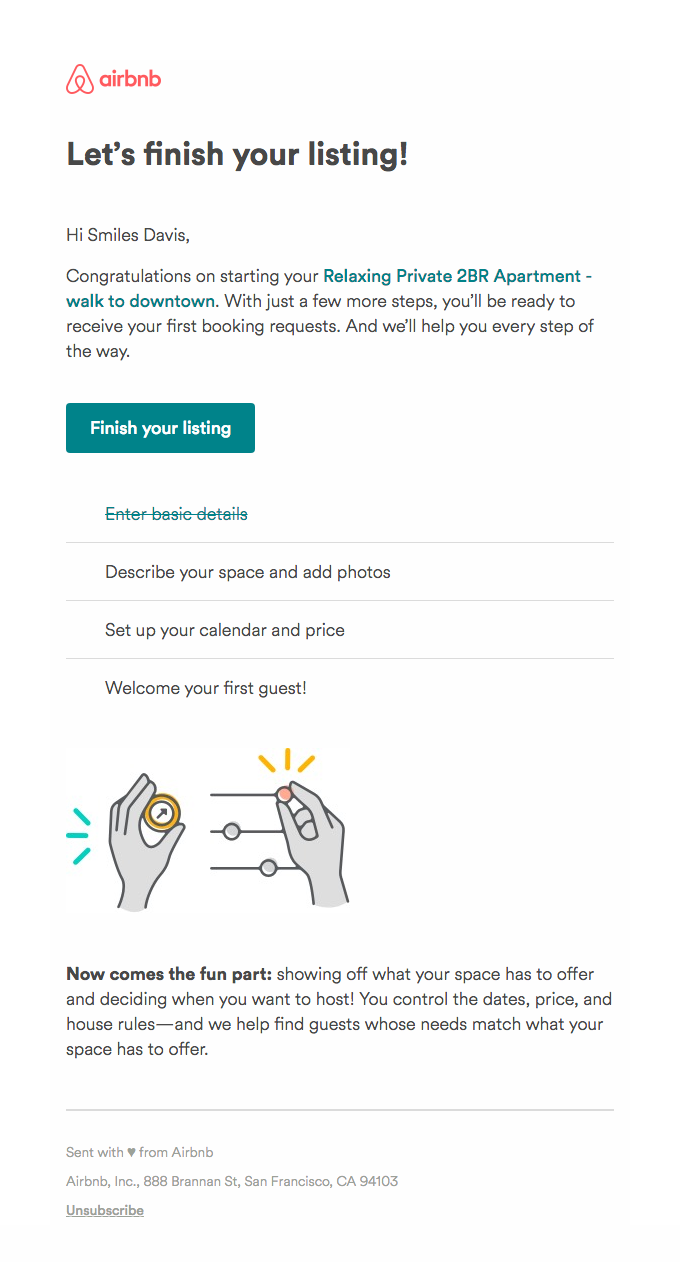This image depicts an advertisement on a website for Airbnb. The prominent elements include the Airbnb logo, consisting of a red lowercase "airbnb" text paired with a red emblem to its left. Bold black letters command attention with the message, "Let's finish your listing!" 

Below, a greeting addresses the user, “Hi Smiles Davis, congratulations on starting your relaxing private two-bedroom apartment walk to downtown. With just a few more steps you'll be ready to receive your first booking requests and we'll help you every step of the way.”

A blue button labeled "Finish your listing" prompts the user to take action. Underneath this, there is a checklist of steps necessary to complete the listing:

1. **Enter basic details** – This is crossed out, indicating completion.
2. **Describe your space and add photos**.
3. **Set up your calendar and price**.
4. **Welcome your first guests**.

Accompanying these steps is a graphic featuring two hands. The left hand holds a yellow or gold compass with an arrow, emitting three lines to the left. The right hand features three sliders: the top one is red and nearly all the way to the right, the second is blue at about 20% to the left, and the third is blue, positioned roughly midway.

At the bottom, a motivational line reads, “Now comes the fun part showing off what your space has to offer and deciding when you want to host! You control the dates, price, and house rules, and we help find guests whose needs match what your space has to offer.”